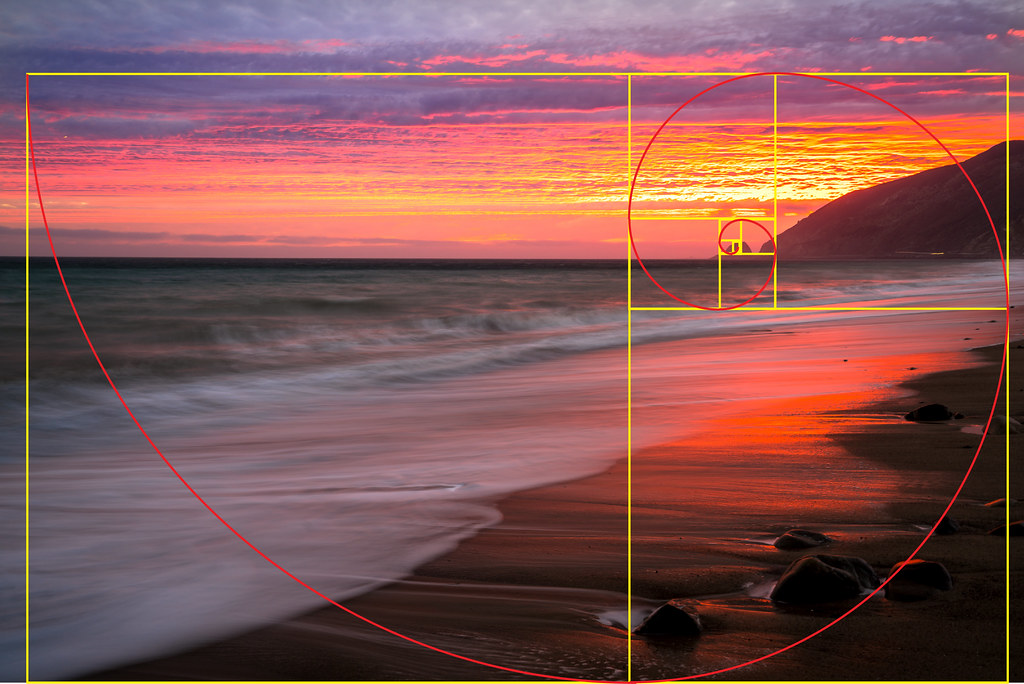This nature photograph captures a serene beach scene at sunset. The coastline stretches along the left side, with calm, flat waves gently reaching and receding from the sandy shore. The sky is a breathtaking palette of orange, red, and purple hues, with wisps of white clouds accenting the top. These vibrant colors are mirrored on the wet sand, creating a glowing reflection. Scattered rocks embedded in the sand are visible in the foreground, adding texture to the scene. The right side features distant mountains that frame the landscape. Overlaying this picturesque view is a large yellow rectangle that nearly encompasses the entire image. Within this yellow frame are several smaller rectangles and squares. A prominent red spiral starts from the top left corner of the large yellow box, curves down to the bottom edge, then winds its way around to make contact with each yellow line it encounters, creating an intricate overlay pattern on the tranquil beach scene.